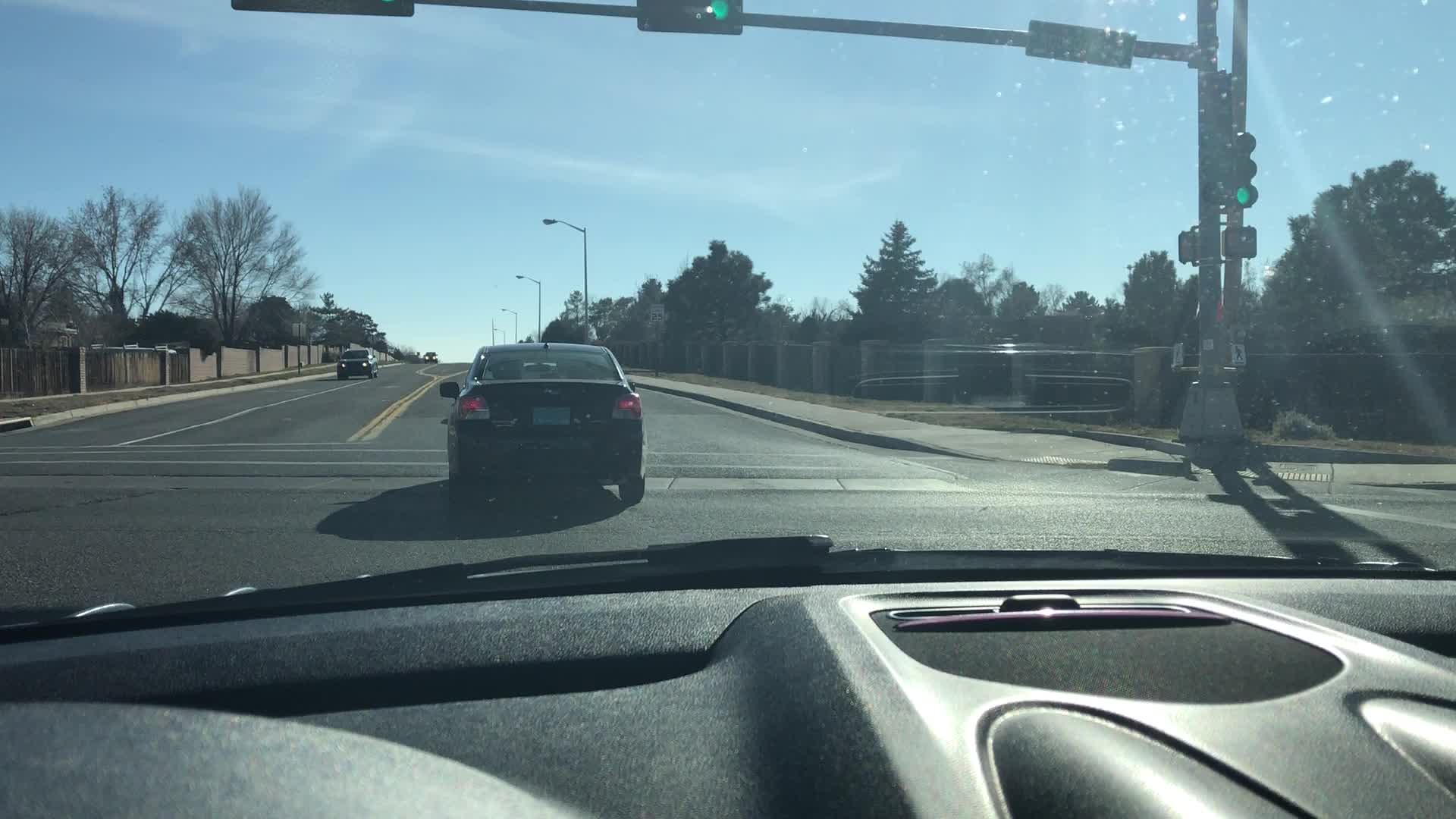The image captured by a dash cam from the driver's perspective appears to be taken inside an American vehicle. Positioned near the steering column, the dash cam view is from the bottom left-hand side of the windshield. In the foreground, there's a small black car, which is undetermined in make and model, progressing through an intersection under a green traffic light. This traffic light is mounted on a pole at the side of the road and extends outwards over the street, clearly visible with its green signal illuminated. On the right side of the image, oncoming traffic is seen traveling down a four-lane road, with two lanes dedicated to each direction. Flanking either side of the road are lush trees, adding a touch of greenery to this urban setting.